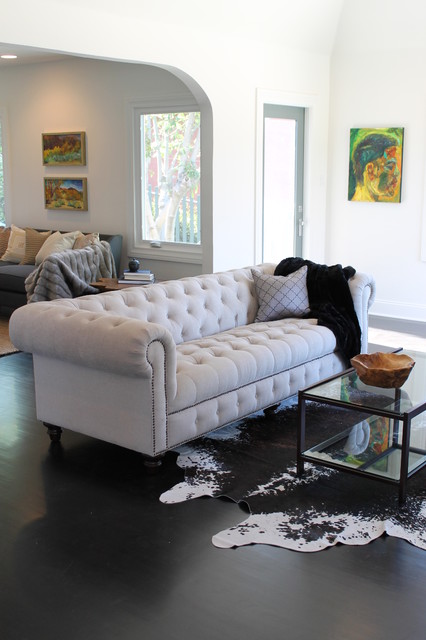This image showcases two adjoining living rooms within a house, connected by an archway. The formal living room in the foreground features a light gray couch adorned with a diamond-patterned pillow and a black throw. It's positioned in front of a glass-topped table with a black metal frame, which holds a wooden bowl for decoration. Below the table lies a black and white cowhide rug on a shiny black floor. The room's stark white walls contrast with a vibrant painting on the far wall, portraying the side profile of a man in green, blue, orange, and yellow hues. To the left of this painting is a door leading outside.

In the background, the second, more casual living room holds a medium gray couch draped with a light gray throw and several white and beige pillows. This couch is placed near a large window that invites natural light and offers a view of the trees outside. Above the couch hang two landscape paintings. The room also features a stack of books and a small decorative item on a table, surrounded by a carpeted floor.